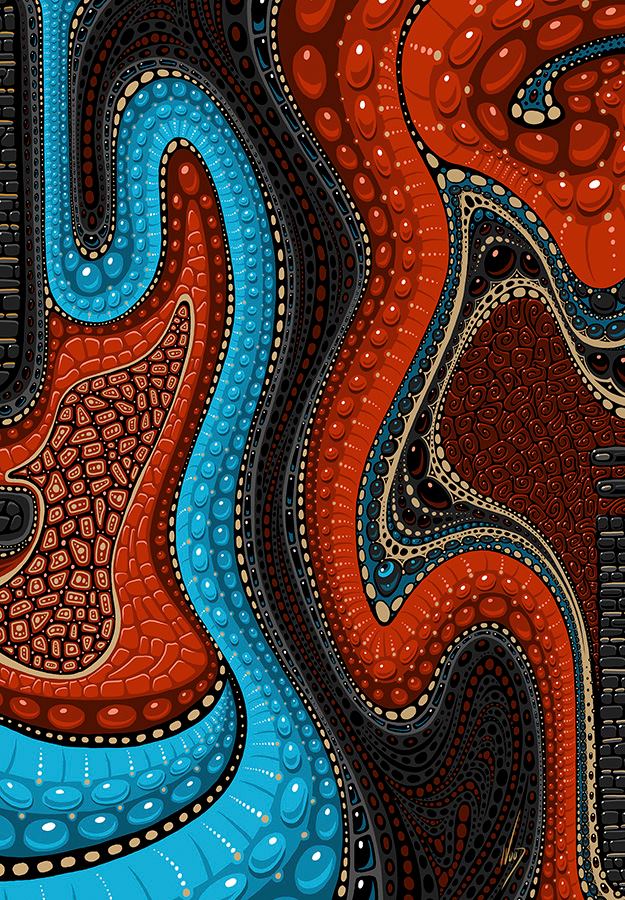This image is an intricate and dynamic piece of abstract art that portrays two guitars intertwined in a yin and yang formation. The guitar on the left is bright blue with a red interior, adorned with circular designs that create a striking and harmonious pattern. In contrast, the guitar on the right is predominantly red with similar circular motifs. The vivid color palette includes bright and medium blues, various shades of red from maroon to deeper tones, as well as burgundy, black, and cream. These colors blend together in a free-form, psychedelic manner reminiscent of mixed oils or flowing, tentacle-like curves. The surface of the image features elements that appear three-dimensional, like high-specular reflections on water droplets or jelly beans, contributing to a shiny and almost wet look. Additionally, parts of the image suggest anatomical forms or textures, such as red spots, black and red streaks, and areas resembling pomegranate seeds. The entire composition is dynamic, with a notable sense of movement and fluidity, showcasing a balance of complementary colors and forms.